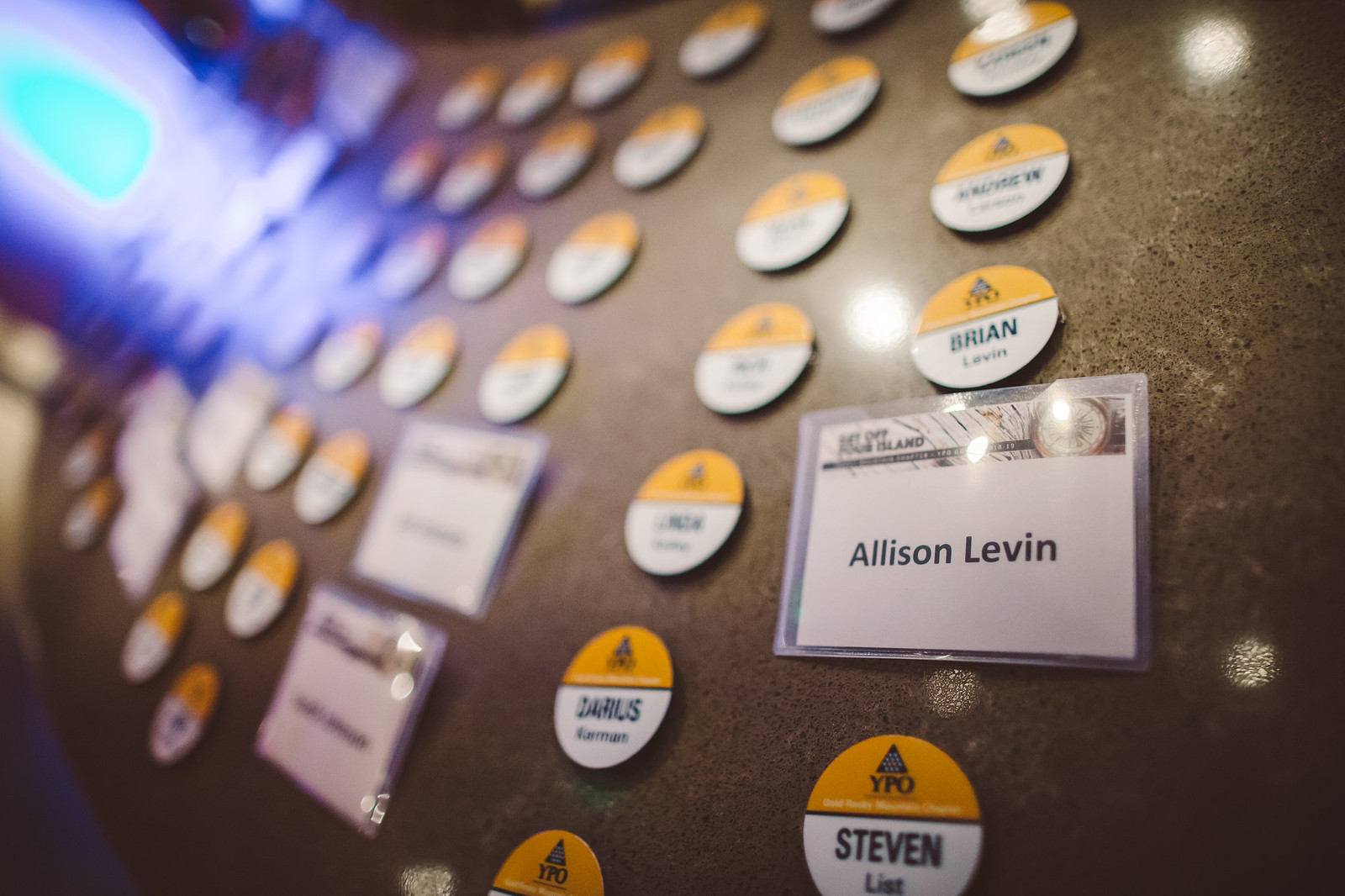The image displays a slightly tilted, fuzzy photograph of a brown marble table speckled with darker brown and white spots. Arranged on the table are several rows of name tags and circular pins, all predominantly featuring a yellow top half and a white bottom half, with black text. Among the visible names on the tags are Brian, Steven, and Darryl on the circular pins, and Allison Levin on a rectangular, laminated plastic tag. Each tag also bears the acronym "YPO," likely indicating the name of the organization. The scene suggests a company event where participants pick up name tags from the table to identify themselves. Various lighting shadows add depth to the image.